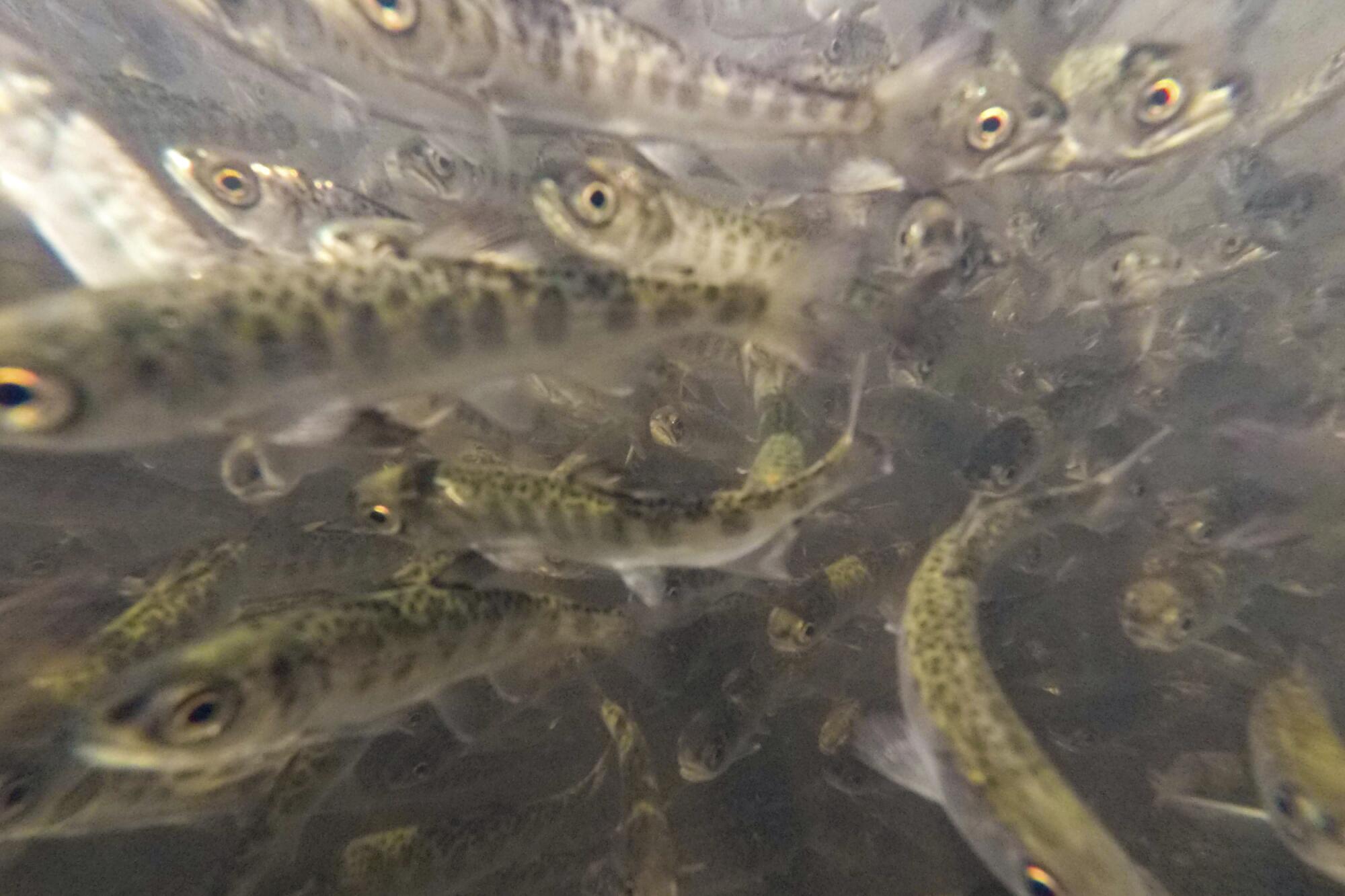This full-color underwater photograph captures a mesmerizing scene of a large school of slim, elongated fish swimming in various directions but maintaining close proximity. The natural light reveals the intricate details of their bodies. The fish, all presumably of the same species, exhibit big, golden-yellow eyes with darker centers that sometimes catch the light, giving them a striking appearance. Their upper bodies are a mix of brown adorned with vertical black patches that resemble thumbprints, while their underbellies are a faint whitish hue. The water surrounding them has a slightly grey, almost magnified look with hints of green seeping through. The background is simply this aquatic environment, enhancing the sense of depth and movement within the fish school. The scene is dense with fish, positioned on the left, right, and even overlapping, creating a dynamic and almost surreal underwater tableau.